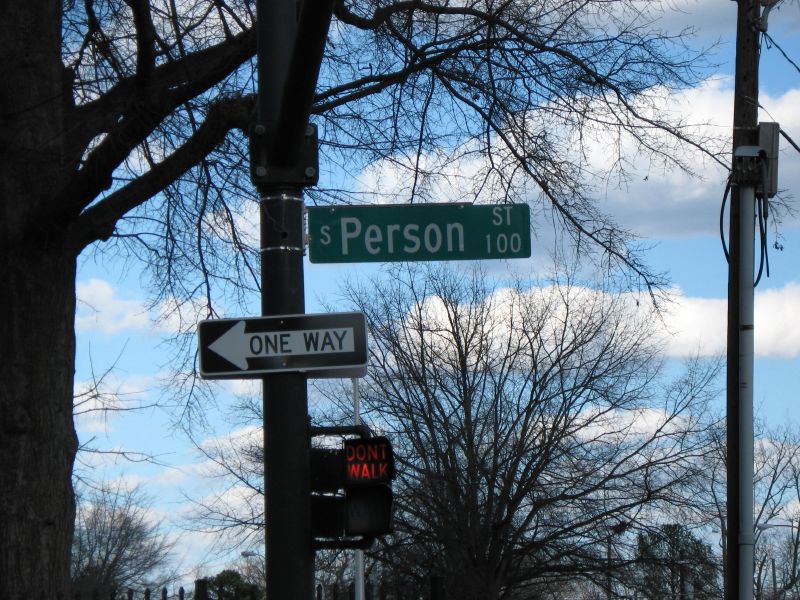This photograph, presented in a rectangular format, showcases a serene blue sky adorned with scattered white clouds as its background. Dominating the left side of the image is the silhouette of a tree trunk, appearing almost black due to the shadows. However, towards the base, hints of gray bark become visible. Thin branches sprout from the lower part of the trunk, while thicker branches extend upwards towards the center top of the photograph.

On the right side, from the upper to lower corner, a steel pole stands prominently. At the top of this pole, electrical wires stretch out and descend towards the right. An electrical box is also mounted at the top, with heavy wires emerging from it.

Centrally positioned in the image is another pole which prominently features a green street sign that reads "South Pearson Street 100 block." Additionally, a black and white one-way sign is attached to this pole. A traffic signal displaying a lit-up "Don't Walk" message is also visible, adding an urban element to the otherwise natural and serene setting.